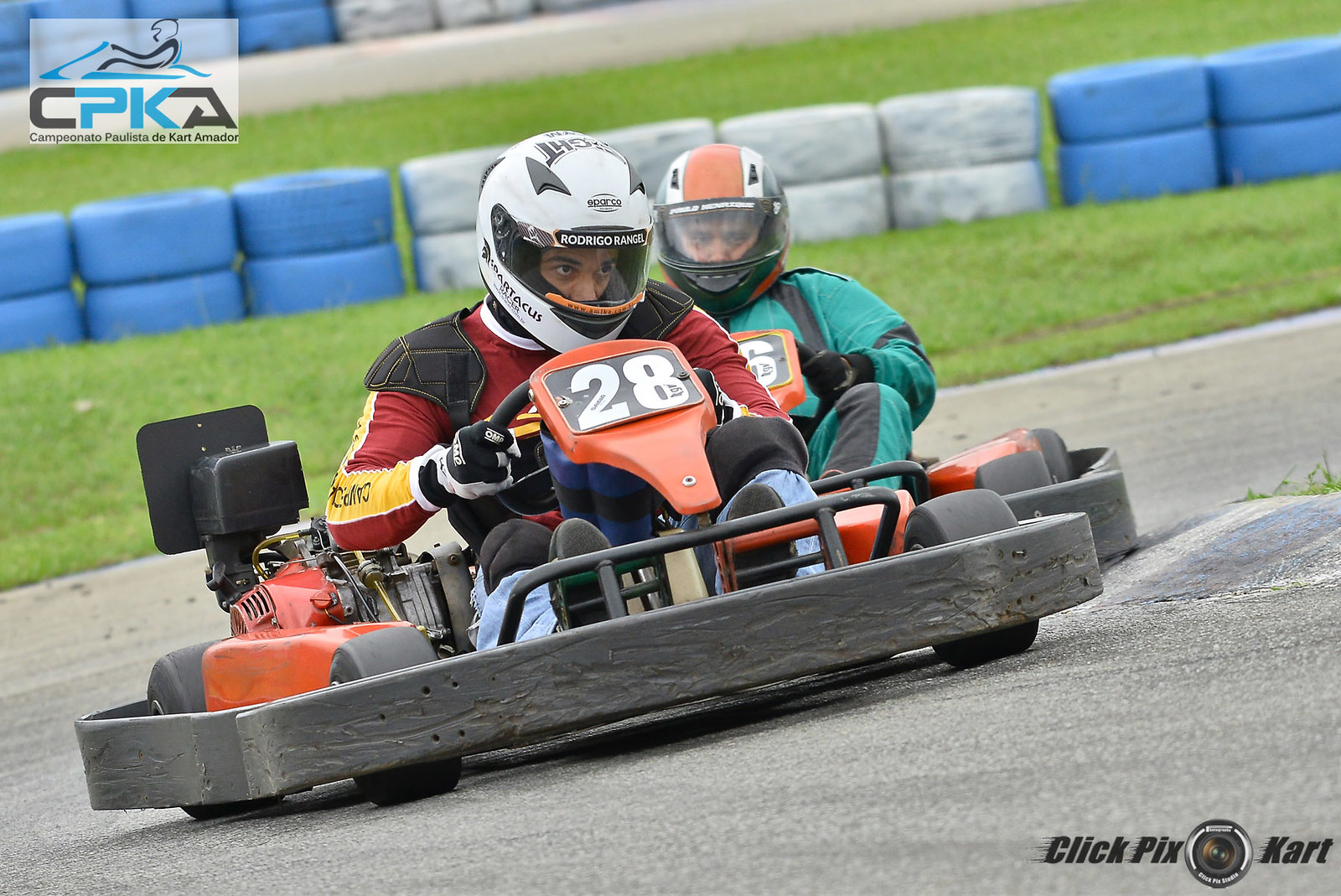This outdoor image captures an intense moment on a go-kart race track, featuring two racers navigating a curve on a concrete course lined with blue and gray tires acting as safety barriers. The prominent racer in the foreground, driving go-kart number 28, is in a vehicle with distinct orange accents and a large gray bumper. He is wearing a white helmet adorned with black markings and the text "Ricardo Ranch," along with a maroon and yellow long-sleeved racing shirt and gloves, firmly gripping the steering wheel. The motor of his go-kart is visibly on the side. Trailing closely behind is another racer clad in green and black coveralls, wearing an orange and white helmet, and driving a similar go-kart. In the top left corner of the image, there is a CPKA logo, while the lower right corner features "ClickPixKart" with a small camera icon. The background shows a grassy area, adding a vivid contrast to the action on the track.